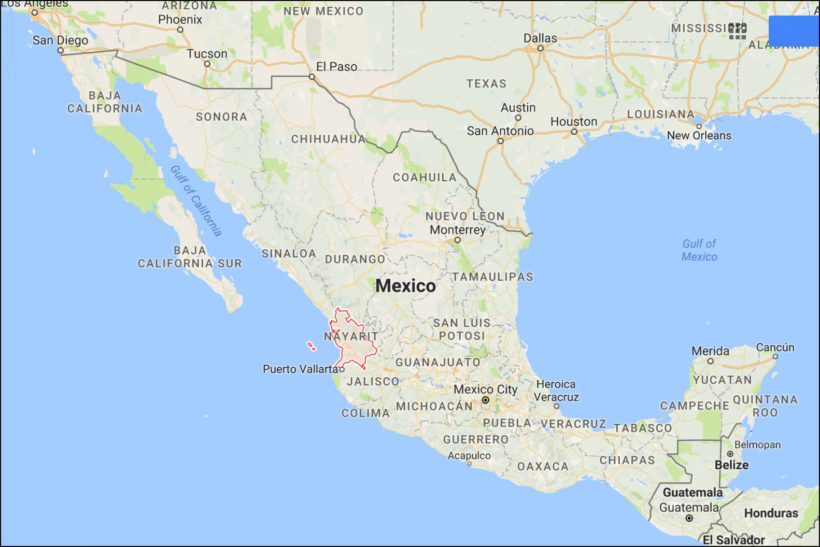The image depicts a detailed map of parts of North and Central America, prominently featuring Mexico and several U.S. states and cities. In the United States, the map highlights El Paso, Tucson, San Diego, and the state of Texas with its major cities: Dallas, Austin, San Antonio, and Houston. It also includes Louisiana and its well-known city, New Orleans.

In Mexico, the map showcases various states and cities such as Baja California, Oaxaca, Chiapas, Puebla, Mexico City, Heroica Veracruz, Colima, and Puerto Vallarta. It also mentions neighboring Central American countries Honduras and Guatemala.

The map features two Baja California locations, possibly indicating the Baja California Peninsula. Above the Mexican region, the map marks the United States. Overall, this image provides a comprehensive geographic overview, detailing significant cities and regions across both countries.